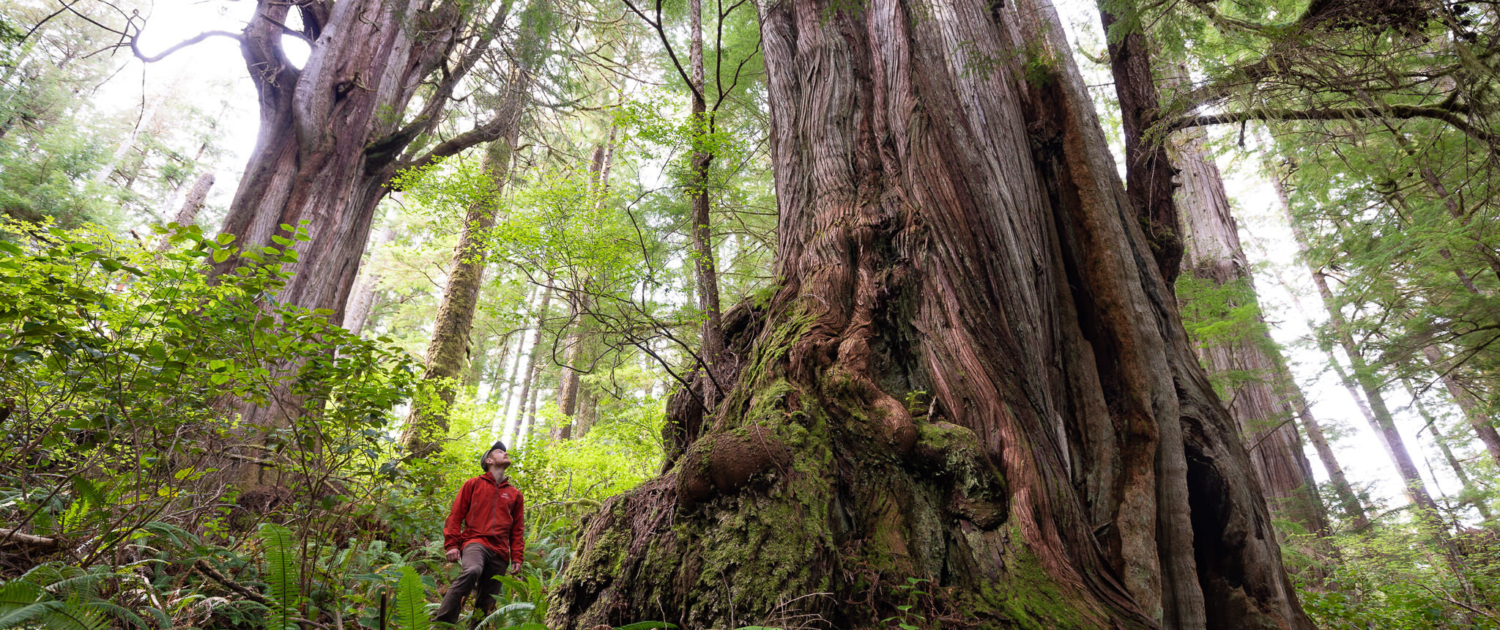In this photorealistic image, we see a person standing in a majestic forest, surrounded by towering trees. The focal point is an enormous tree with a large trunk, possibly a California redwood, covered in ridges and green moss at the base. The person, dressed in a red jacket, gray pants, and a hat, is looking up in awe at this giant tree. The person appears small next to the immense trunk, which could be centuries old. The forest is filled with lush greenery, numerous thinner trees, and saplings. Some of the smaller trees have white trunks, adding contrast to the vibrant scene. Sunlight filters through the canopy, casting a light and ethereal glow throughout the woods, accentuating the natural beauty of the scene.